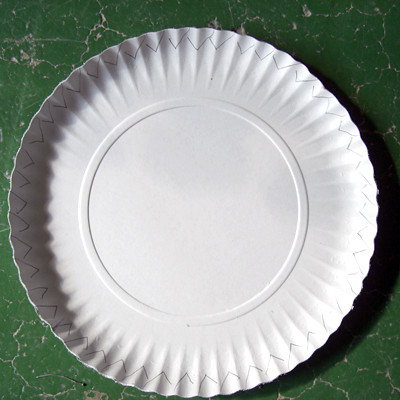The close-up image features a white paper plate with a distinctive raised circle in the center and a patterned, folded edge, suggestive of cheap, easily bendable paper plates. The plate's edges are decorated with small, gray, V-shaped lines creating peaks. It sits atop a green, marble-like table, characterized by light gray cracks and chips that bleed through the painted surface. The plate, nearly touching the photo's top edge, casts a prominent shadow due to the bright lighting, particularly noticeable on its left side. The overall palette of the image is primarily white and green.